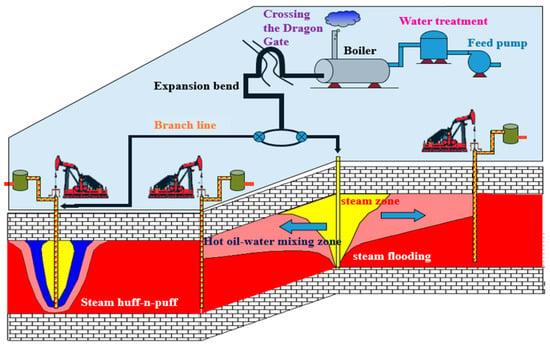The image features a highly detailed, partially schematic diagram that depicts a complex industrial process, potentially related to oil drilling or wastewater treatment. The diagram is divided into an underground section filled with red hues to signify heat and multiple labeled zones. At the bottom, the "Hot Oil Water Mixing Zone," "Steam Zone," "Steam Flooding Zone," and "Steam Huff and Puff" zones are illustrated, with each having distinct passages leading upward. These passages connect to several pumps and piping systems above ground. 

The surface level showcases a series of interconnected components, starting with a boiler, leading to water treatment, followed by a feed pump, and then an expansion bend. The layout also includes a notable feature labeled "Crossing the Dragon Gate." The components are depicted as basic cylindrical shapes with tags, and the entire setup gives a cartoonish impression with brick textures and a blue background.

Despite the thorough depiction of each part, the overall purpose of the diagram remains somewhat ambiguous, though it likely represents a simplified model of an oil drilling operation or a similar industrial process.